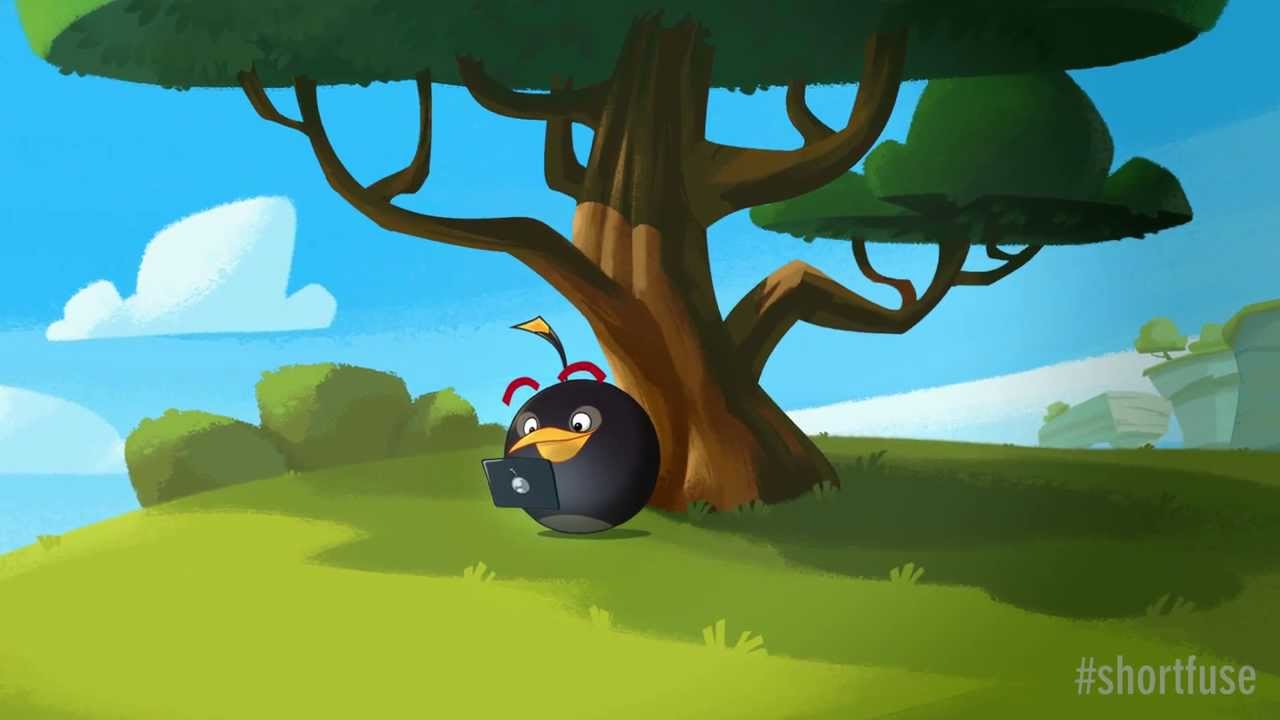This is a digitally created graphic cartoon set outdoors during the daytime, featuring a single, bird-like character seated under a tree. The character is a round, black ball with a gray base, adorned with an orange bill, two eyes, red eyebrows, and a yellow feather-like tip on its head. The character appears to be looking down at or holding a black tablet with a gray logo on the back.

The tree, positioned centrally in the image, has a sturdy brown trunk branching out into three main limbs, all covered in clusters of green leaves. The surrounding grass in the foreground varies in shades from lime green to pea green and dark green, with sunlight illuminating the left side while casting shadows on the right.

To the left of the character are three bushes, and in the backdrop on the right, there are rocky cliffs with additional trees. Above, the blue sky hosts a few scattered white clouds. The entire scene is overlaid with the text "#shortfields" in the bottom right corner, written in a transparent white font. The image is in a landscape layout, with the top and bottom edges longer than the sides.